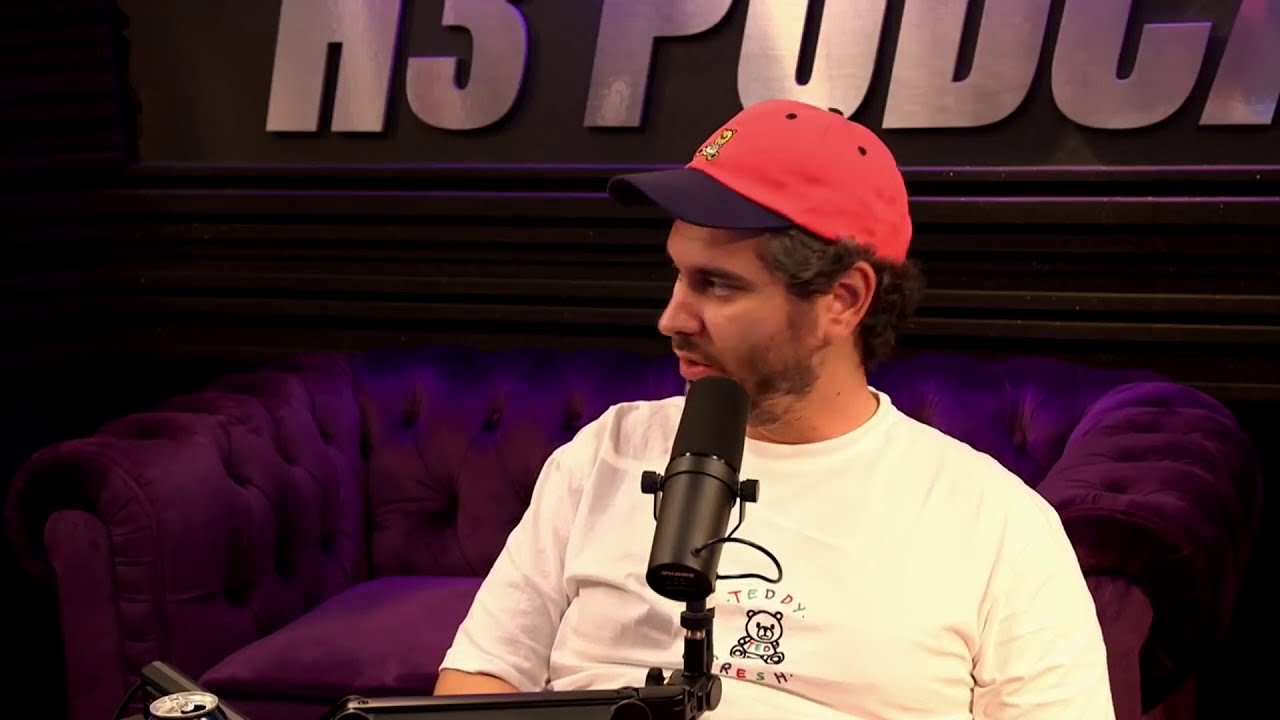This image is a screenshot from the H3 Podcast show, featuring a man as the main focus, seated slouched backwards in front of a professional articulable microphone. He is wearing a red baseball cap with a dark brim, showcasing curls of his dark, thick hair peeking out from beneath the cap. His face is adorned with a scruffy beard and mustache, giving him a slightly rugged appearance, and he has a tan complexion. He is dressed in a white t-shirt with the center displaying the words "Teddy Fresh" and an illustrated bear labeled "Ted" between the text. A barely visible open can of soda can be seen at the bottom right corner of the screen. The backdrop features a plush, purple velvet tufted couch, with part of the H3 Podcast logo in silver displayed on a wood-paneled wall behind him.